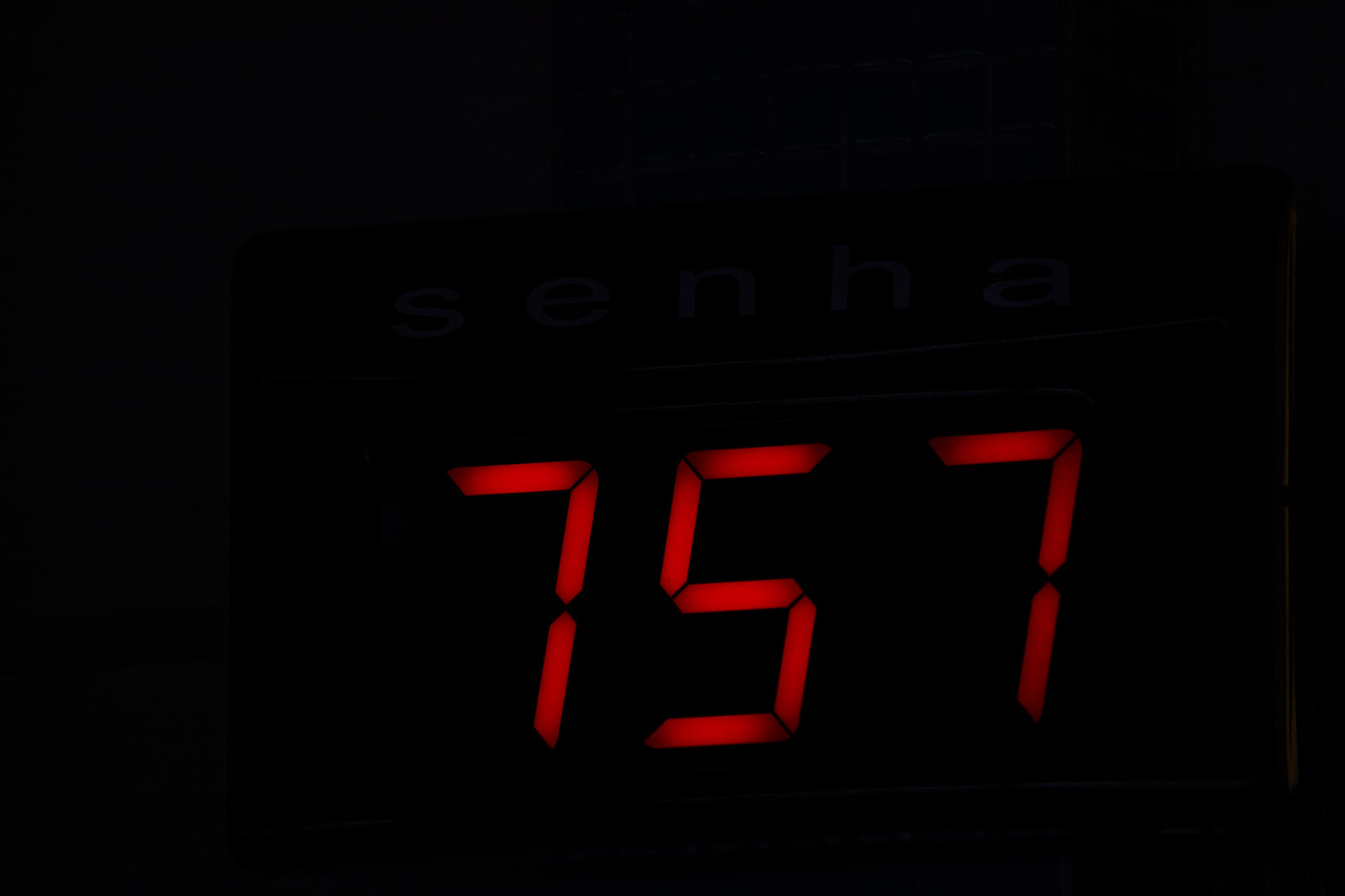This photograph, although of very poor quality, appears to capture the faintly illuminated face of an older digital clock. Despite the extreme dimness and overall blackness that pervades the image, you can make out the disjointed outlines of red digits in the bottom right center. These digits, which seem to be fading at their join points, read "757." This suggests the time displayed is 7:57, though the clarity and illumination are significantly compromised.